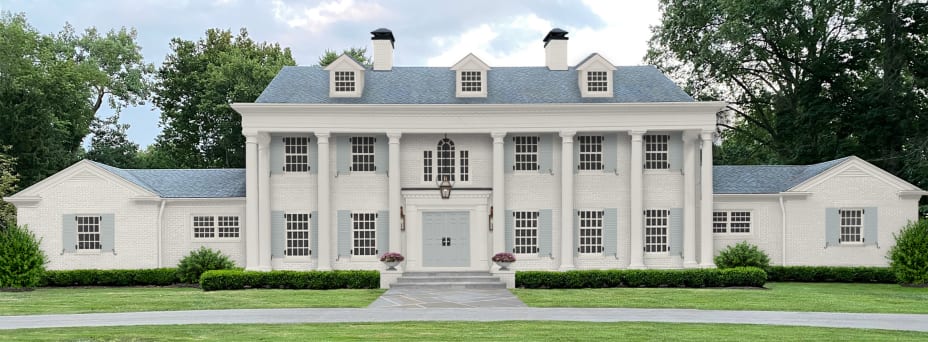This is a detailed, outdoor daytime photograph of a grand, plantation-style manor. The central section of the house is two stories tall, featuring a striking white facade and a brownish-blue roof with three dormer windows extending out, each capped with blue gable roofs. The entrance is framed by a set of six to seven grand white columns that support the roof, giving the home a classical architectural aesthetic.

The main double door is gray and accented with an arched window and two sidelights, topped with a light fixture. Two chimneys stand tall on either end of this section. The windows are large, consistent across both stories, and divided into smaller panes, adding to the traditional charm. A small porch at the front is complemented by flower pots on either side of the stairway that leads to this central entrance.

On either side of the main building are one-story wings, also white with gray gabled roofs, echoing the style of the central structure. A manicured lawn stretches in front of the house, bordered by a set of hedges and a tiled marble walkway leading to the entrance. The clear blue sky with scattered white clouds serves as a picturesque backdrop, accentuating the overall elegance of this grand estate. While the image has a highly detailed, almost render-like quality, its visual portrayal is clear and striking, capturing the allure of this expansive, classically styled home.